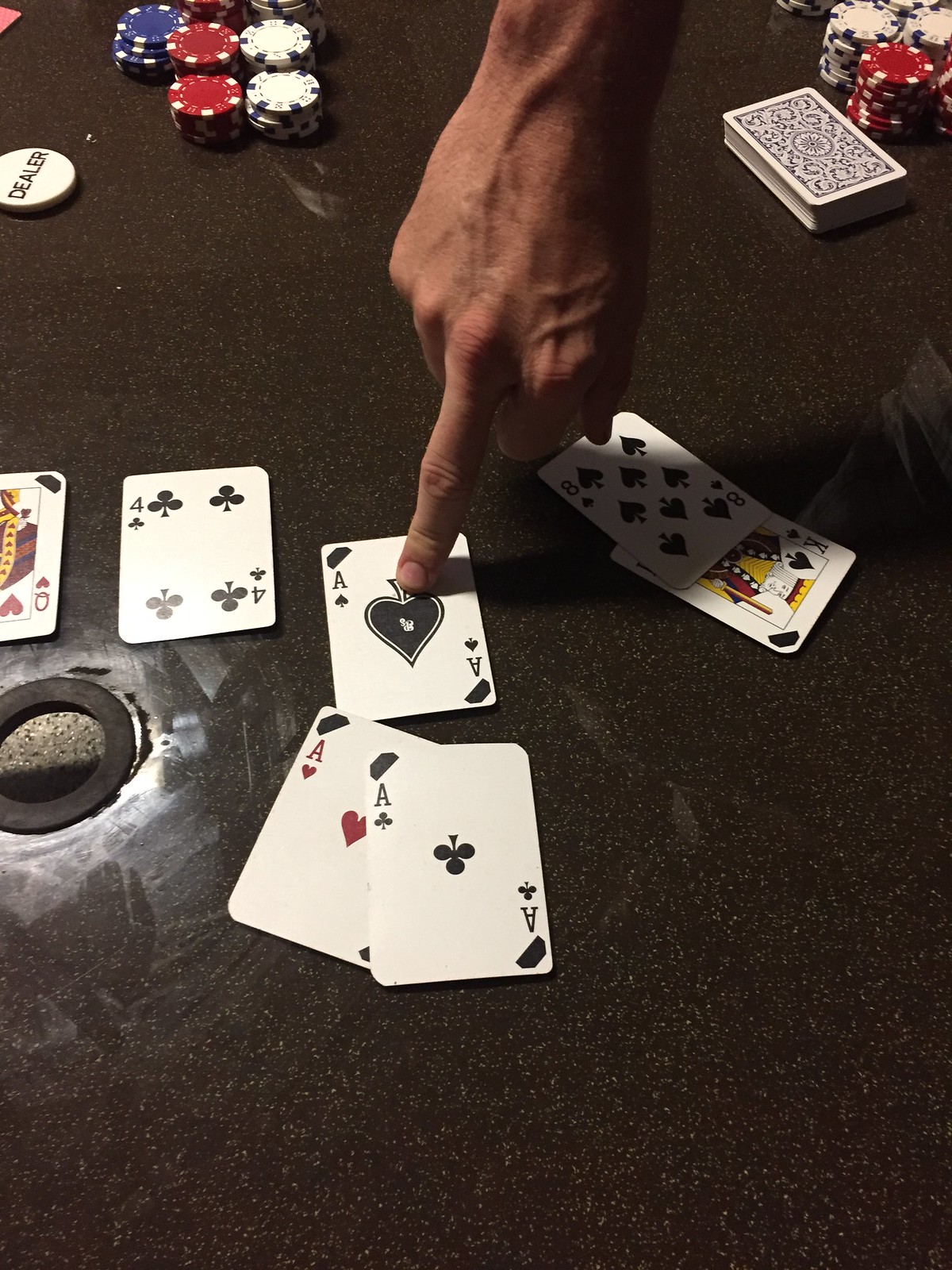This detailed photograph captures an intense moment during a card game, set in an indoor environment with a table that intriguingly appears to be designed for outdoor use due to the central hole typically meant for an umbrella. The tabletop is black with a sparkly, high gloss finish, adding a touch of elegance to the scene.

In the upper left corner, a white dealer chip with black lettering clearly spells out "DEALER." A visible array of poker chips is meticulously arranged: a stack of blue chips, two stacks of red chips, and two stacks of white chips to the left, while the upper right holds an additional two stacks of red chips and two stacks of white chips next to a neatly positioned deck of cards.

Attention is drawn to the center of the image by a man's hand, prominently featuring his middle finger touching an ace of spades card. The table displays an intriguing mix of cards: a four of clubs, ace of spades, ace of hearts, ace of clubs, six of clubs, eight of clubs, and a king of spades, hinting at a captivating hand in play. The overall composition vividly captures the tension and excitement of the card game, set against an unexpected yet stylish backdrop.